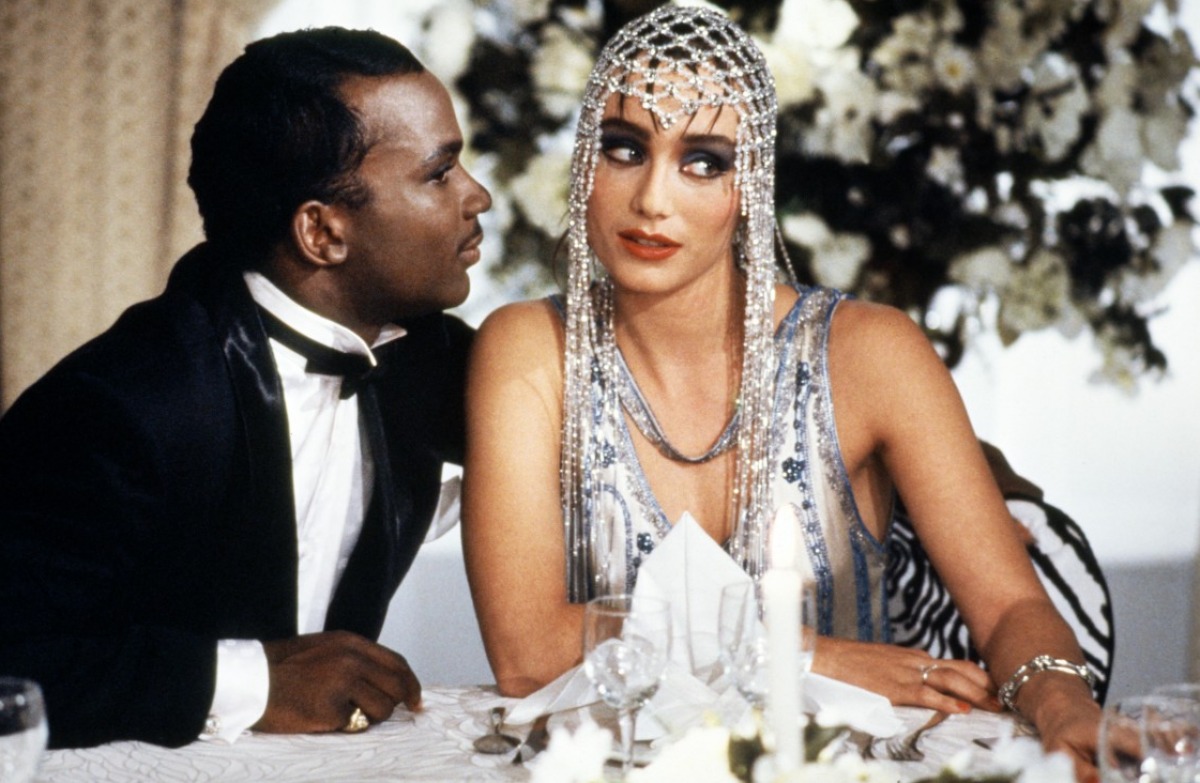The photograph features an elegantly dressed African-American man and a white woman seated at a classy dinner table. The man, positioned on the left, is leaning in towards the woman as if whispering into her ear. He is attired in a black tuxedo with a bow tie, and a gold ring adorns his right pinky finger. The woman, dressed in a silver-blue silky gown with a strap hanging down from her neck, has her head adorned with a beaded headdress. She is wearing dark eyeshadow, mascara, and red lipstick, and her hands are decorated with various pieces of jewelry, including a ring on her right hand and a bracelet on her left. The table is covered with a white tablecloth, and is set with wine glasses and intricately folded white napkins. In the background, a bouquet of flowers and some indistinct trees add to the upscale ambiance of the setting.